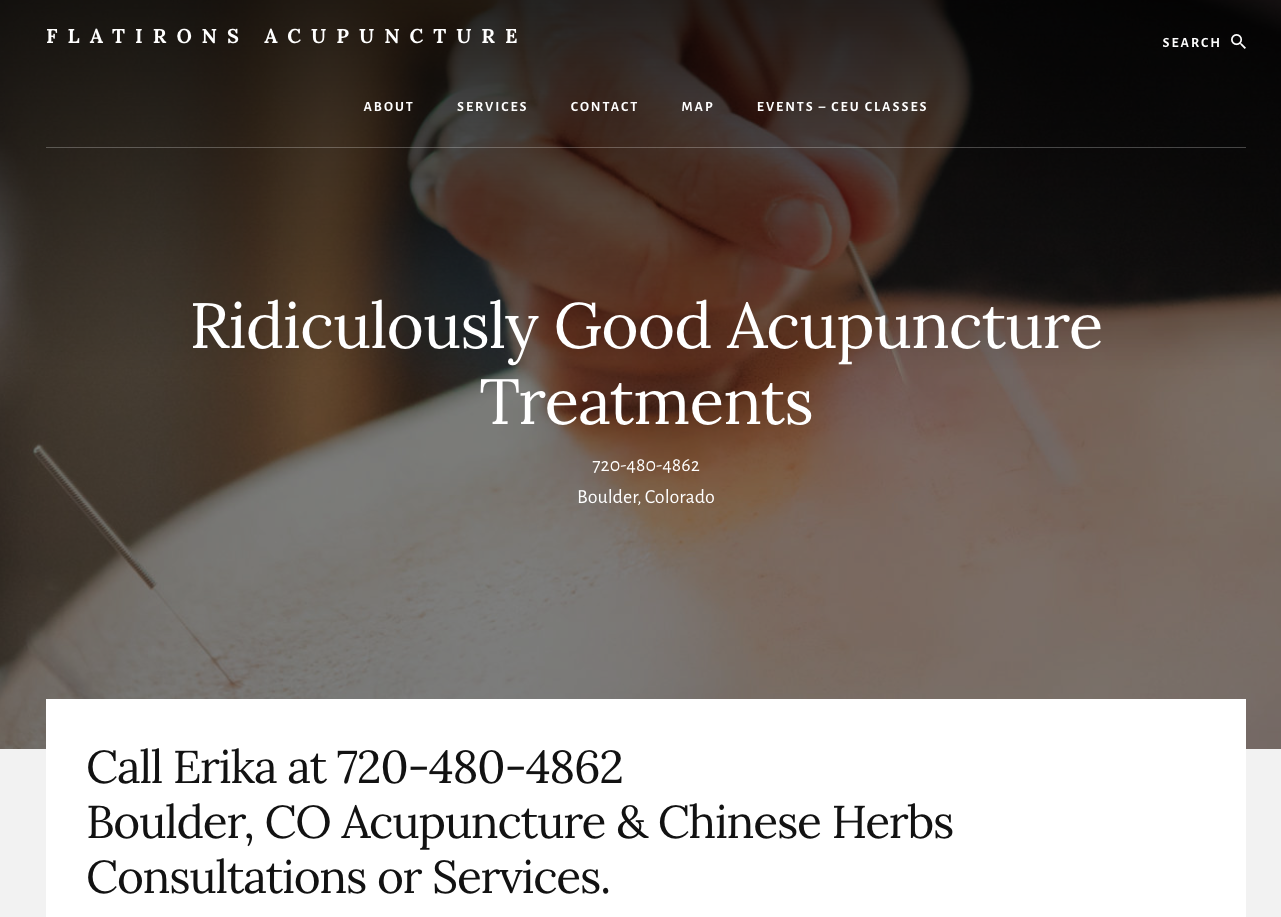This is a screenshot of a website for Flatirons Acupuncture. The website features a close-up background image of a tanned Caucasian woman's hand inserting needles into skin, which has a dark overlay to enhance text legibility. The website's name, "Flatirons Acupuncture," is prominently displayed in white text in the top left corner. To the right, there is a search bar with a magnifying glass icon. Just below the site name is the main navigation menu with links labeled About, Services, Contact, Map, Events, and CEU Classes.

The center of the screen showcases the tagline "Ridiculously Good Acupuncture Treatments" in a serif font, accompanied by the contact number 720-480-4862 and the location Boulder, Colorado. At the bottom of the image is a white rectangle with black text that reads, "Call Erica at 720-480-4862, Boulder, Colorado, Acupuncture and Chinese Herbs, Consultations or Services."